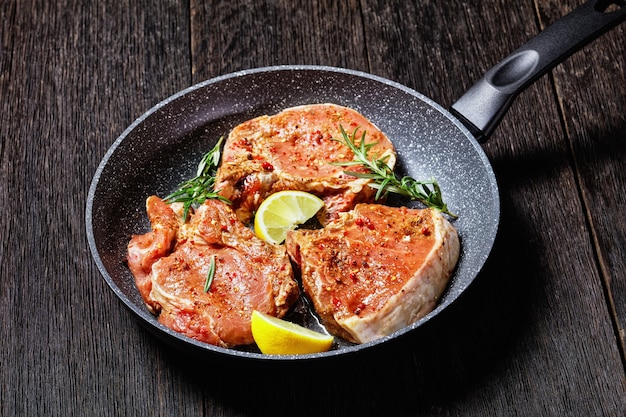The image depicts a frying pan resting on a dark wooden table comprised of four vertically oriented planks. The pan itself features a black surface speckled with white and has a black plastic handle extending towards the upper right corner, complete with a thumb indentation. Inside the pan are three generously seasoned, thick cuts of meat, likely sirloin steaks or possibly beef or pork. These are adorned with a liberal application of red spices, obscuring the meat beneath. Accompanying the meat are two lemon slices, one situated in the middle and the other in the lower portion of the pan, along with sprigs of green herbs—possibly rosemary—positioned on either side.